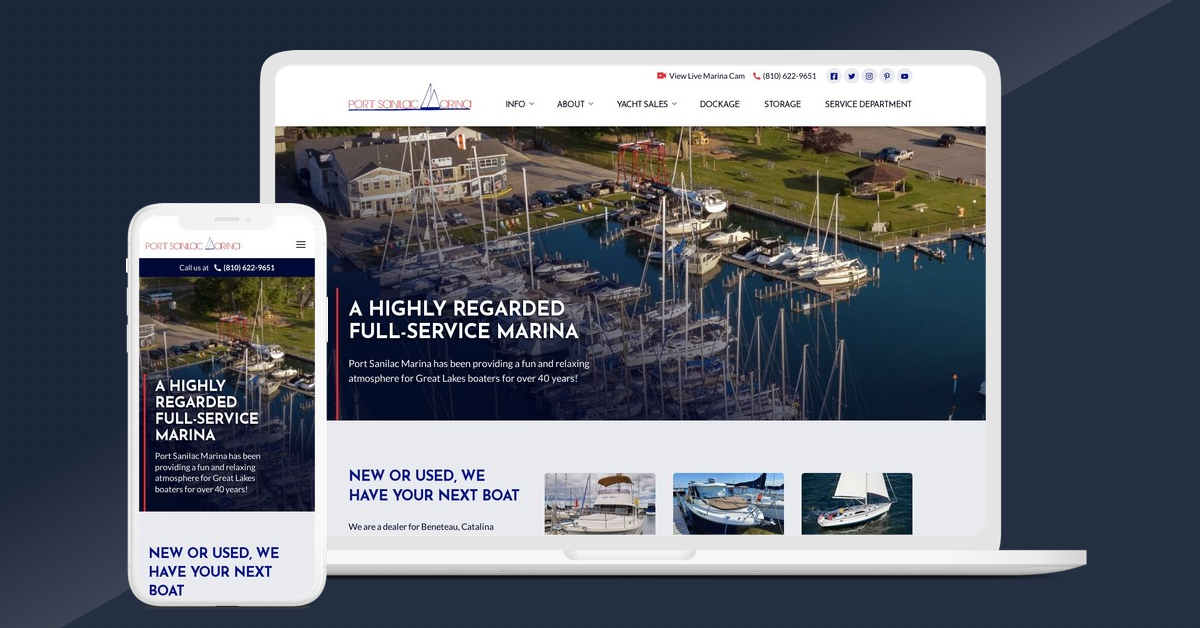The screenshot showcases a responsive website displayed on both a laptop and a smartphone. The website features a prominent image of a bustling dock or port filled with various ships and boats. The headline on the main page proclaims the marina as "a highly regarded full-service marina." Below this, a tagline reads, "New or used, we have your next boat." Accompanying this text are images of three distinct boats: the first appears to be a luxurious yacht, the second is unspecified but clearly displayed, and the third boasts a large white sail. The visual layout highlights the website's emphasis on offering a range of boating options suitable for diverse customer needs.